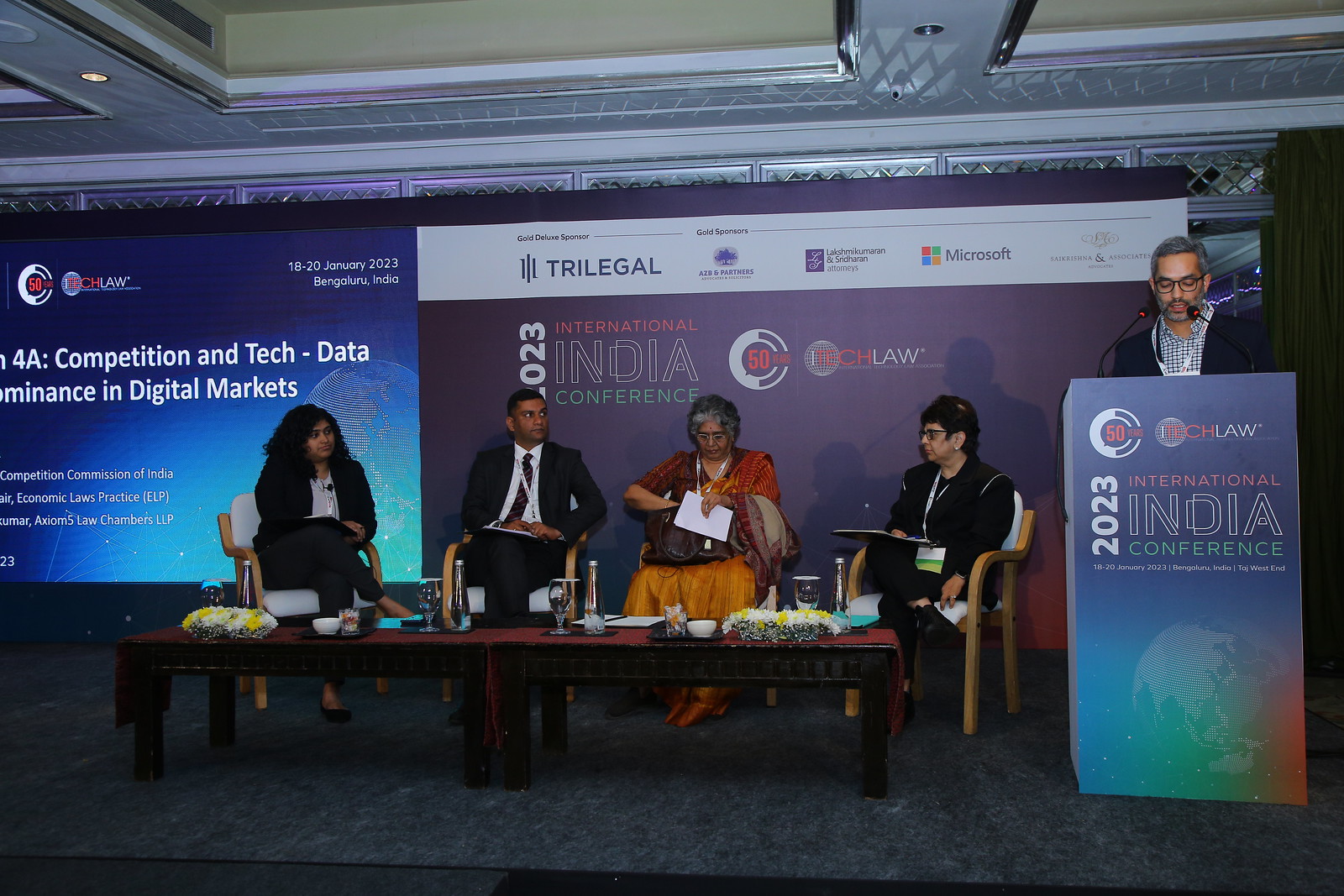The photograph captures the scene of the 2023 International India Conference. The setting is an indoor room with a green ceiling and white bordering. Center stage, a man stands at a podium labeled with "2023 International India Conference," addressing the audience. To his left, four individuals are seated at a long, reddish wooden table, which holds several drinks, including a water bottle. The seated group, all dressed in smart clothing, comprises three women and one man. One woman wears a black outfit, another is in an orange dress, and another is in an all-black suit with a gray shirt, along with a microphone. The man alongside them is in a black suit with a white collared shirt and a black tie. Behind this group is a digital screen displaying details about the conference, including tech, digital markets, and legal discussions, with specific dates from January 18th to 20th, 2023. The backdrop is predominantly purple, featuring the "2023 International India Conference" title and listing the sponsors such as Trilegal, AZB and Partners, Lakshmikumaran and Sridharan Attorneys, Microsoft, and Sakharshina and Associates. The image portrays a formal and professional conference atmosphere with a strong focus on technology and digital markets.